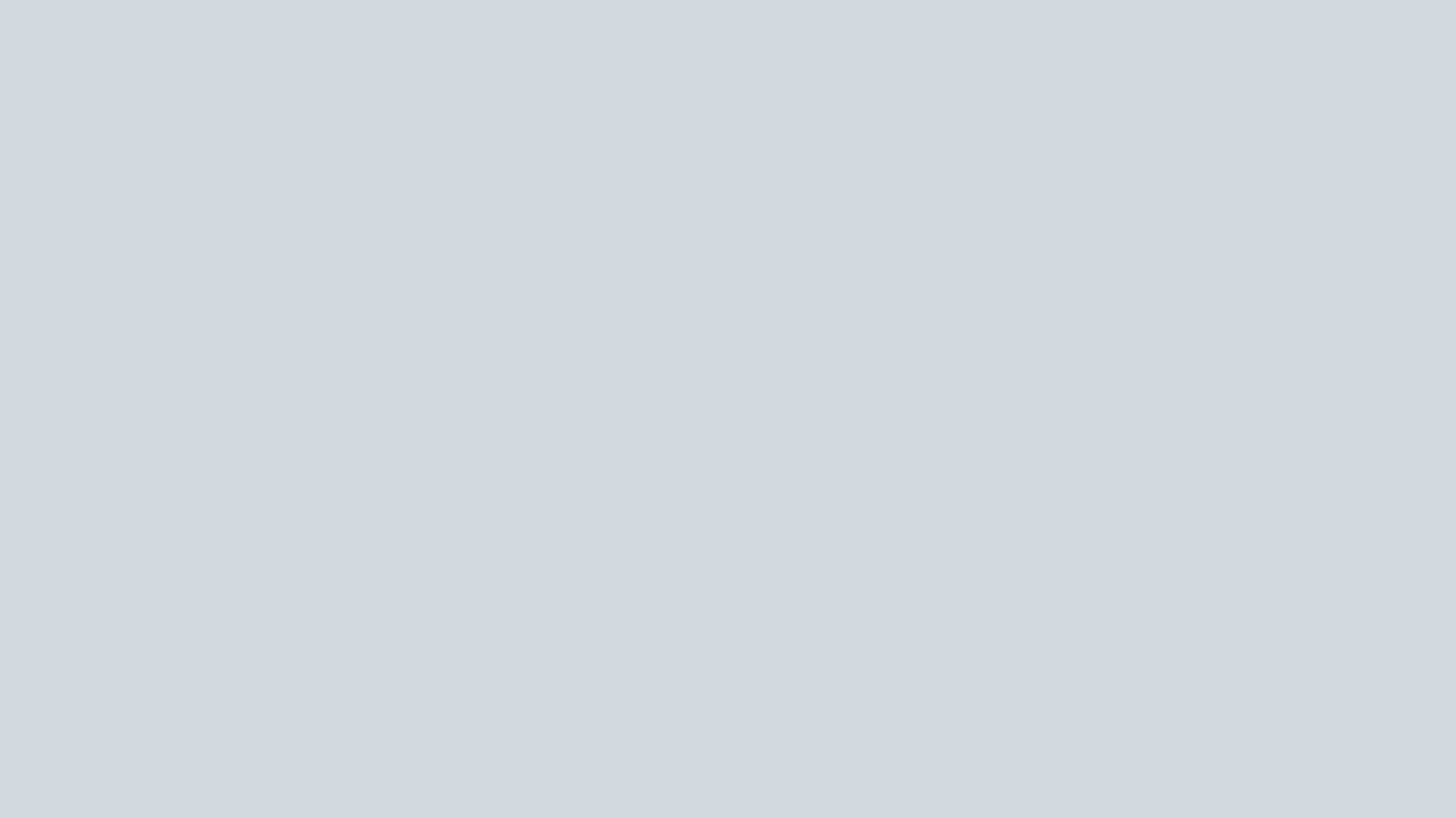A monochromatic image featuring varying shades of grey, devoid of any distinguishable patterns or figures, offering a uniform and seamless grey appearance throughout the entire frame. This minimalist composition emphasizes the simplicity and subtlety of the grey color palette, capturing a serene and understated visual experience.